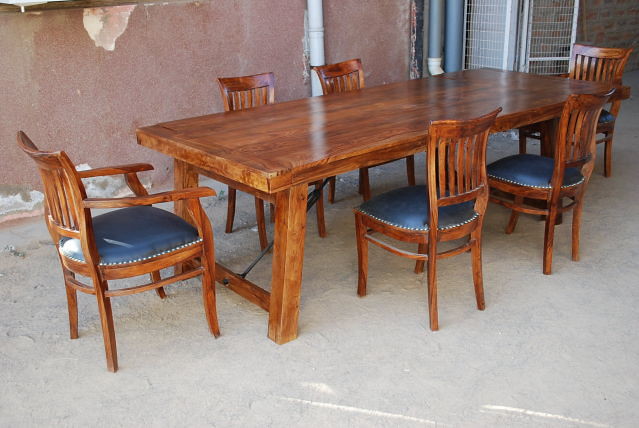The photograph showcases a stunning handmade, polished wood dining table, exuding a rich reddish-brown hue. This massive piece is detailed with robust legs and reinforced with a steel support beam angled beneath, featuring an iron turnbuckle for added stability. Surrounding the table are six exquisitely designed chairs, matching the table's wooden finish. The chair seats are a beautiful greenish-gray, adorned with perfectly spaced tacks around the padding. Notably, the arrangement includes two armchairs, positioned at either end of the table, with the rest sporting elegantly bent wood backs that form small rectangular patterns.

The setting, appearing to be an entryway, features a simple concrete floor and walls plastered in a fading pink paint. These walls, though in need of repair, add a raw, rustic charm to the scene with exposed patches and embedded pipes. Against one wall, there are what seem to be two single bed frames with mattress springs propped up, contributing to the room's eclectic backdrop. Despite its dilapidated surroundings, the focal point remains the beautiful craftsmanship of the dining table and chairs.